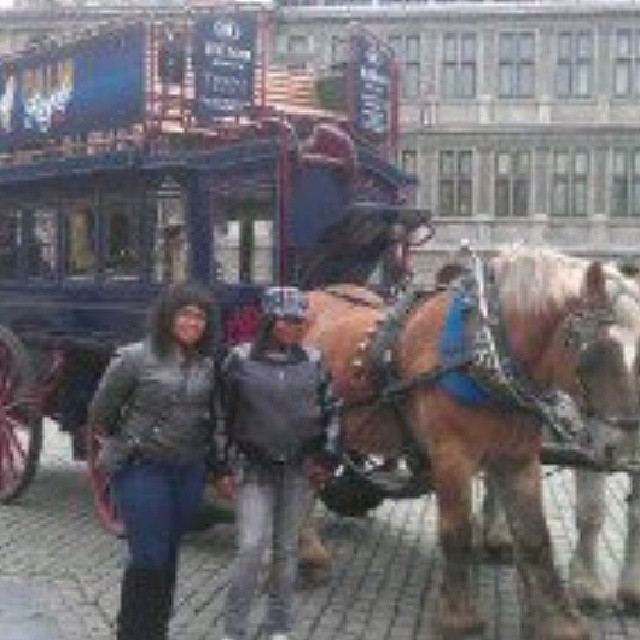The photograph, albeit very blurry and out of focus, captures a busy outdoor scene likely in a touristic area. In the background, there's a building approximately three stories high with many different windows. The foreground features a cobblestone walkway where a brown horse with white hair pulls a large, navy blue double-decker carriage with prominent red wheels. Beside the horse, stand two women of African descent, dressed in black jackets and wearing blue and gray jeans respectively; one of them is also wearing a hat. Though their faces are hard to discern due to the image’s low quality, they appear to be posing and smiling for the camera. Additionally, there are indications of a second horse, likely white or gray, visible only by its legs.